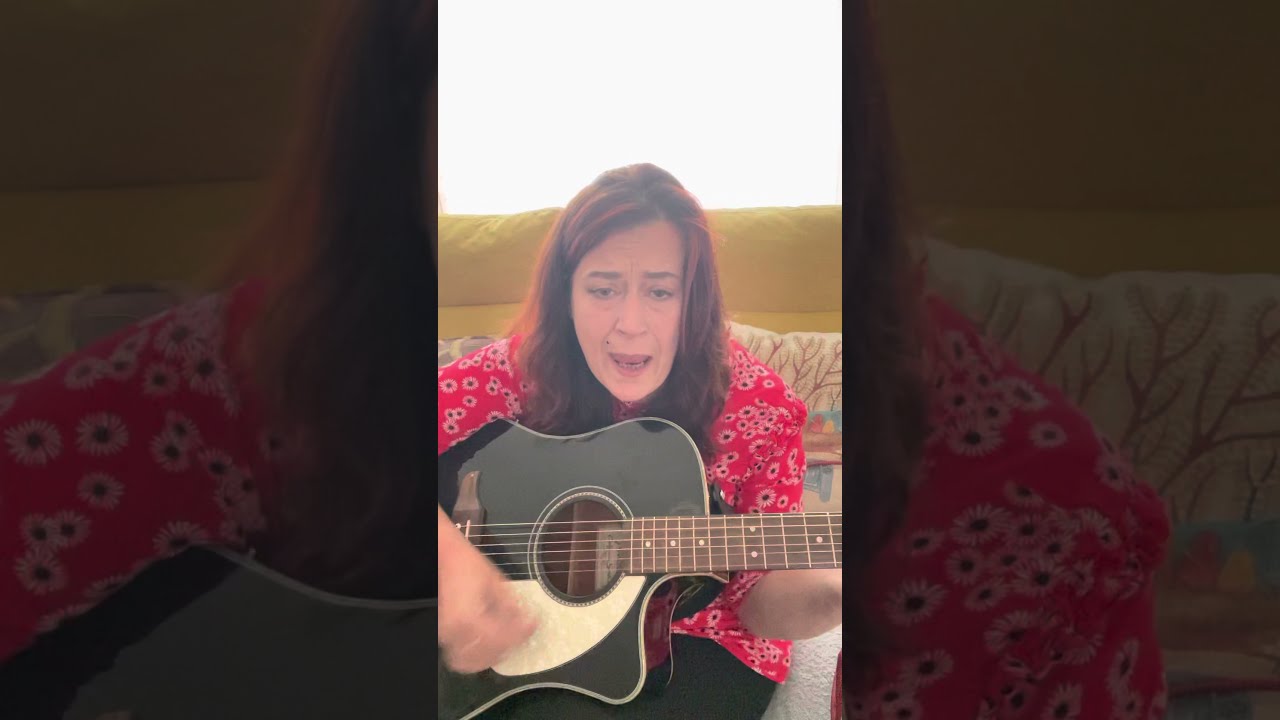The photograph captures a woman in her early 50s, with long brown hair, sitting on a sofa adorned with tree-like patterns on the cushions. She is playing a black guitar, her right hand plucking the strings. The woman wears black slacks and a bright red blouse decorated with daisy-like floral patterns. She has noticeable wrinkles, a beauty mark, and heavy eyebrows, adding character to her serene, yet slightly sad expression as she sings with her mouth open. The background includes a yellow cushion or wall, and behind that, a bright light source, possibly a window, floods the space with sunlight. The image appears to have a border created by blurring and graying out parts of the middle image, enhancing the overall focus on the woman and her guitar.